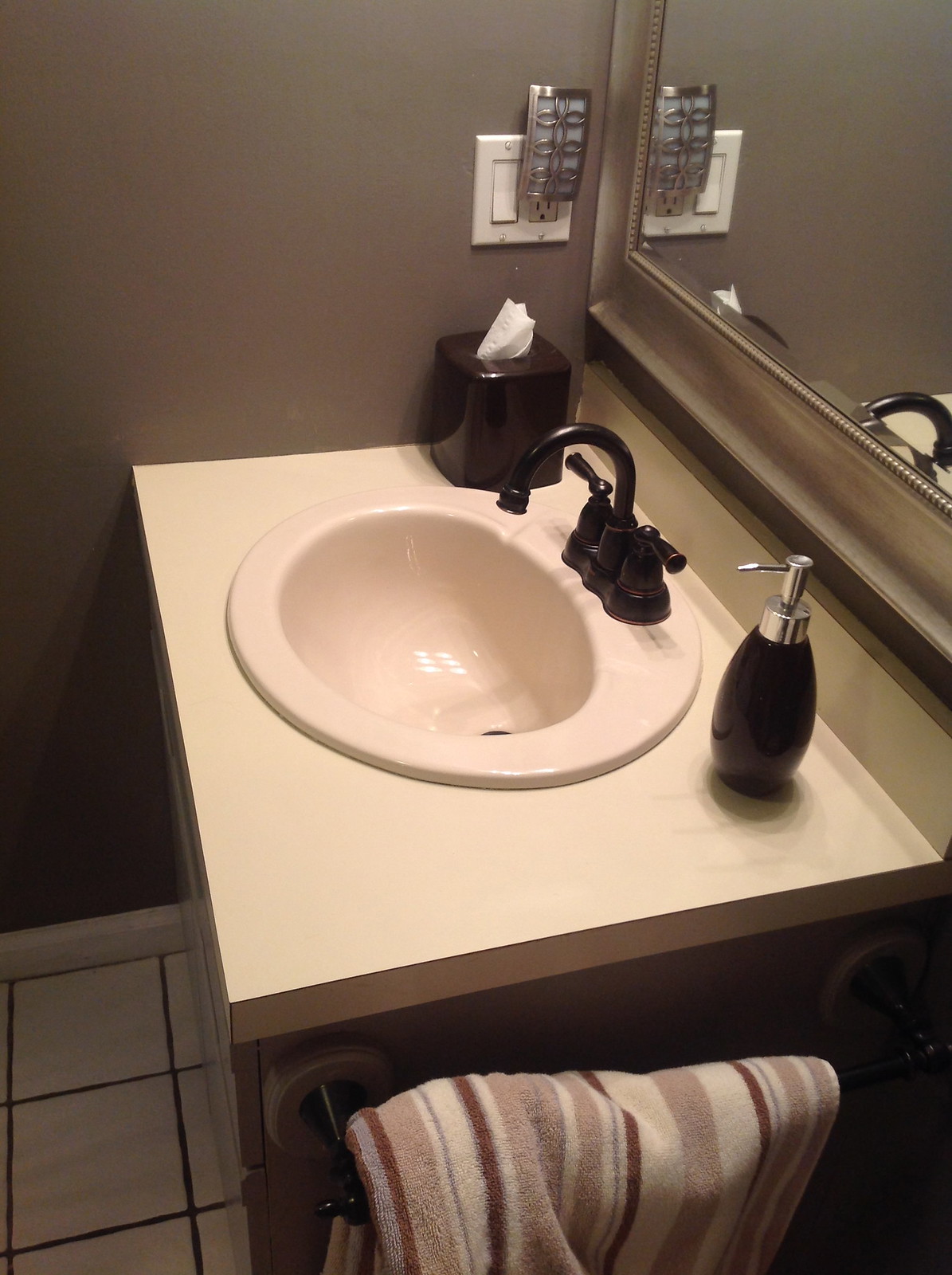This photo captures a modern bathroom, with a clean, minimalist design. Central to the image is a sleek sink featuring a white laminate bowl complemented by a stylish black faucet. To the left of the sink, a gray wall curves around, drawing attention to a rectangular mirror above, framed in a dark, decorative finish with a subtle texture. 

Underneath the mirror, affixed to the sink's counter, is a black decorative tissue box cover on the left side. On the right side of the counter stands a foam soap pump. A striped towel, featuring dark brown, light brown, and cream tones, hangs neatly below the right side of the sink, providing a touch of warmth and texture.

The white tile floor peeks into the frame, adding a crisp, clean aesthetic to the space. Adjacent to the left side of the sink, an outlet embedded in the wall supports a switch and a nightlight, contributing functional detail to the design. Just beneath the mirror, a four-inch backsplash in the same dark, decorative finish extends above the counter, creating a visually cohesive look that ties the elements of the bathroom together seamlessly.